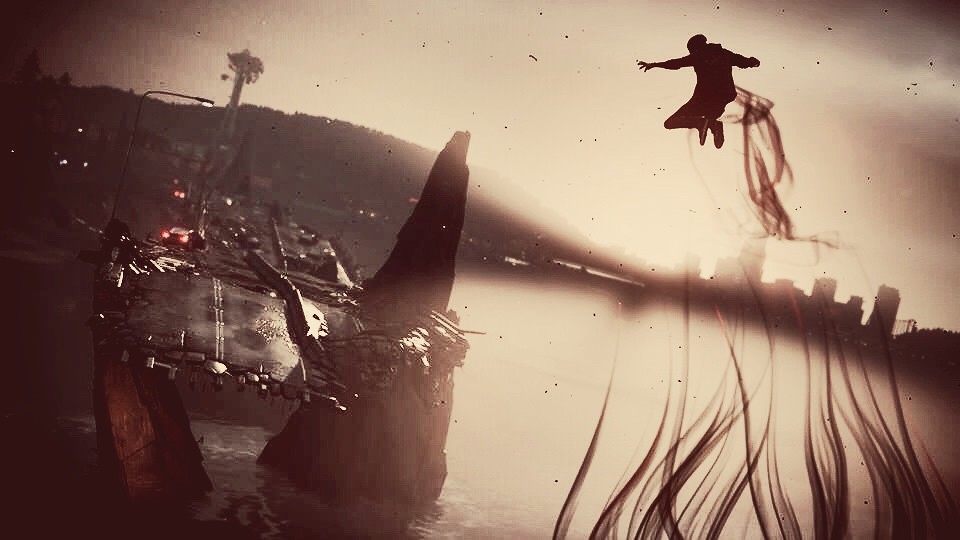This is a screenshot from the video game "inFamous Second Son." The image showcases a dynamic scene where a character, identified by his mid-air leap at the top right, leaves behind a trail of smoke, indicative of his superpowers. This 'rocket jump' propels him towards the lower left quadrant of the image. In this bottom left area, a destroyed and broken road is visible, littered with rocks and various surface anomalies resulting from superpower-induced damage. Additionally, several cars are stranded on the damaged road, their red taillights clearly visible against the chaotic background.